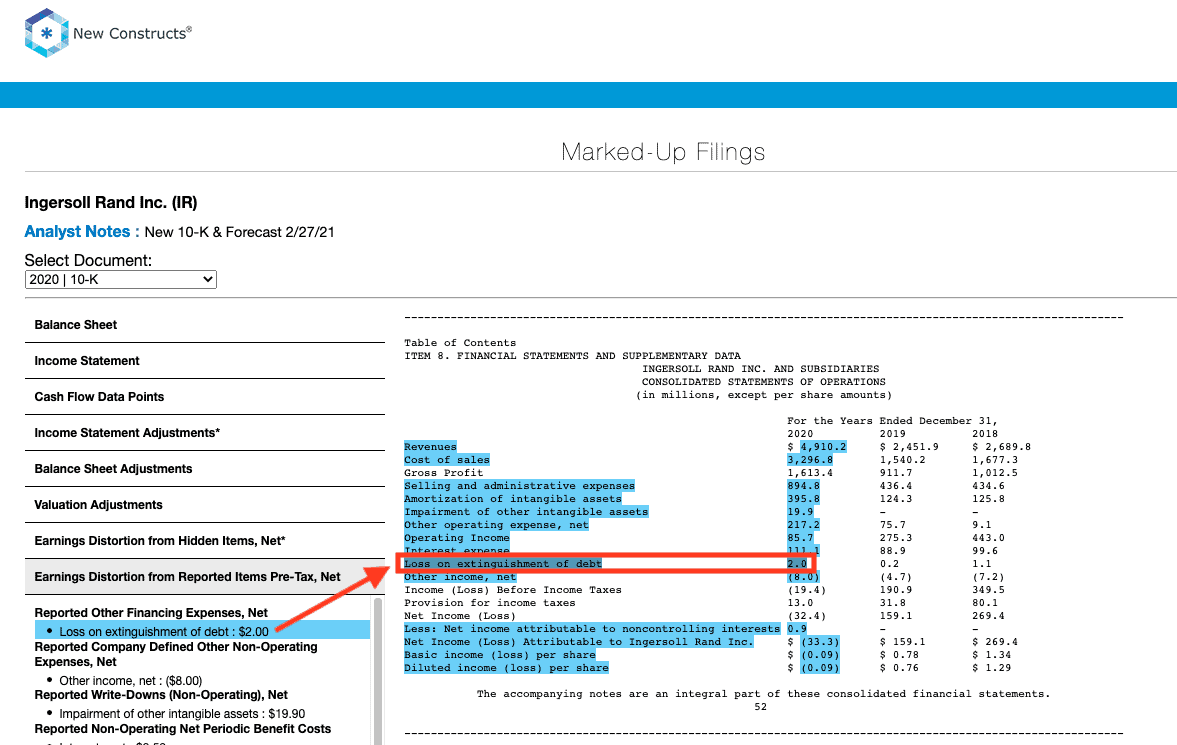The image features a prominent blue logo with varying shades, forming a hexagon shape with a star in the center. To its right, the text "New Construction" is displayed, followed by a blue bar that reads "Mark-Up Filings." Below this, a gray line separates the sections, under which there are several lines of black text, some of which are illegible.

Further down, there is a mix of blue and black text, with a directive that says "Select Document." This is accompanied by a gray-outlined rectangle containing numbers and a downward-pointing arrow. Below this, a series of seven line items in black text are each underscored by black lines, though the specific words are unreadable.

A gray rectangle with more black text, which cannot be identified, is positioned beneath these items. The second line in the list is highlighted in blue, and a red arrow extends from it, pointing to the upper right. Additional black text appears under this highlighted section.

On the right side of the image, a dashed line divides the space, leading to more black text and what appears to be a chart. Much of the chart is highlighted in blue, with a distinct section outlined in a red rectangle where the red arrow is pointing. 

Thank you for watching!